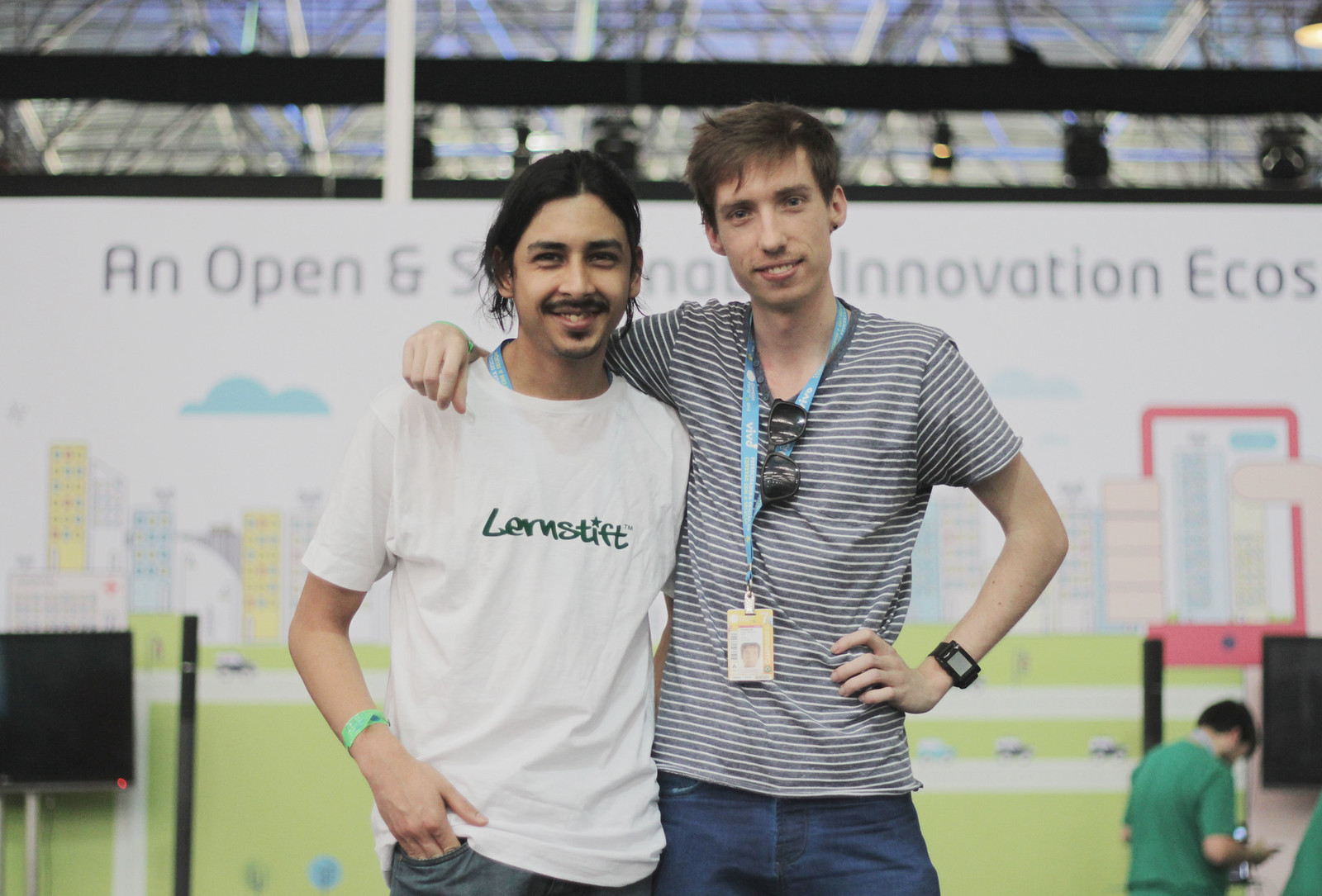The photograph captures a pleasant outdoor scene featuring two men standing side by side and smiling at the camera. The man on the left, who appears Hispanic, has long, dark hair, a mustache, a goatee, and is wearing a white shirt with green text that reads "lernstift." He also sports a green bracelet and a pair of jeans. The man on the right, slightly taller with short brown hair, is wearing a thin black and white striped shirt, a blue lanyard, a watch, and has glasses tucked into his shirt. He has his arm affectionately draped over the shoulder of the man on the left. In the background, a man in a green shirt faces away from the camera, and above him, a large white banner with black text reads "an open innovative ecosystem."